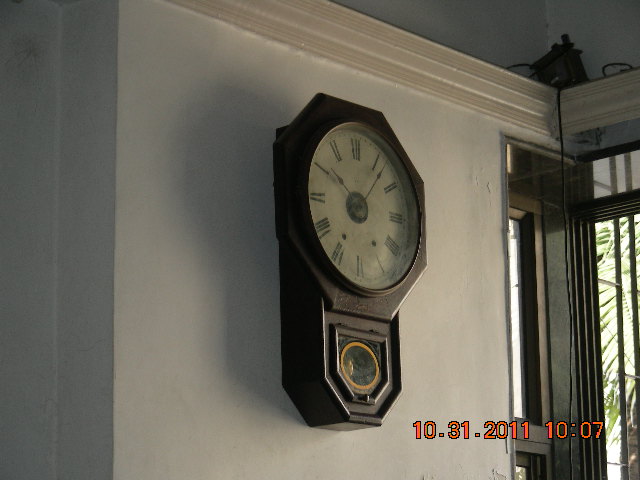The photograph captures a detailed view of a wall clock in a house, specifically a grandmother's clock, mounted on the wall. The clock is characterized by its wooden octagonal frame, intricately crafted with eight sides. The clock face is adorned with finely detailed black Roman numerals marking each hour from one to twelve. The time on the clock is approximately 10:07, as indicated by the shorthand pointing slightly past the 10 and the longhand just past the 1. Additionally, the lower right-hand corner of the photograph features a timestamp reading "10-31-2011, 10:07" in small orange text, which accurately corresponds to the time shown on the clock.